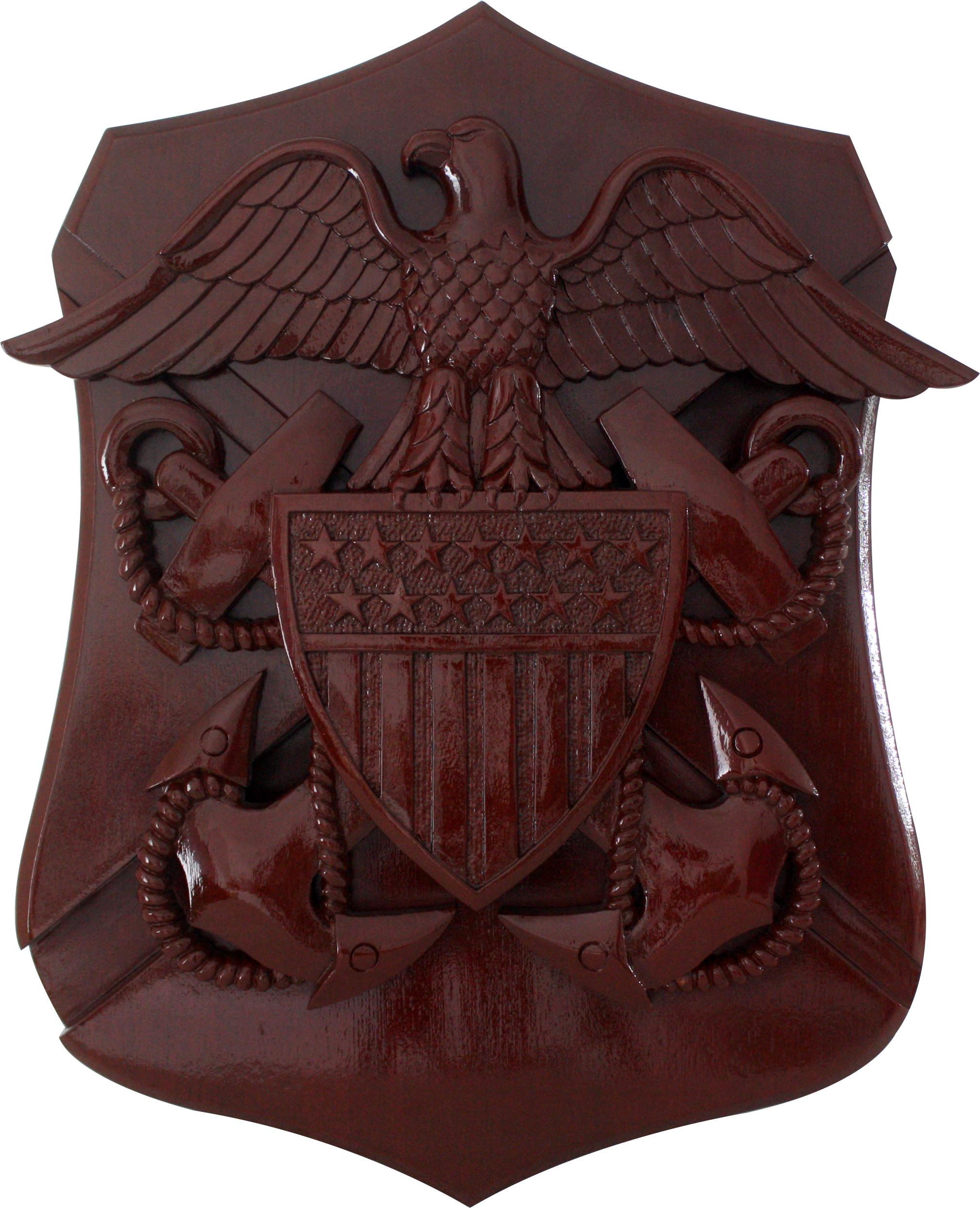The photograph showcases a detailed woodcarving with a highly polished, deep brown finish accented by rich red undertones. This intricately designed plaque appears to serve a military or maritime purpose, featuring a prominent eagle with its wings spread wide at the top. The eagle sits atop a triangular shield that represents the American flag, adorned with 13 stars in two rows—seven stars on the upper row and six stars below—symbolizing the original colonies. The shield also includes six vertical stripes running the length of it. Flanking the shield on both sides are symmetrically placed ship anchors with metal rings at their tops and ropes that wrap around their bases. The overall design is reminiscent of a badge, with the eagle lending a somewhat cartoony but noble appearance. This woodcarving, void of any text or lettering, exudes a sense of historic symbolism and craftsmanship in its elaborately cut grooves and placement of imagery.